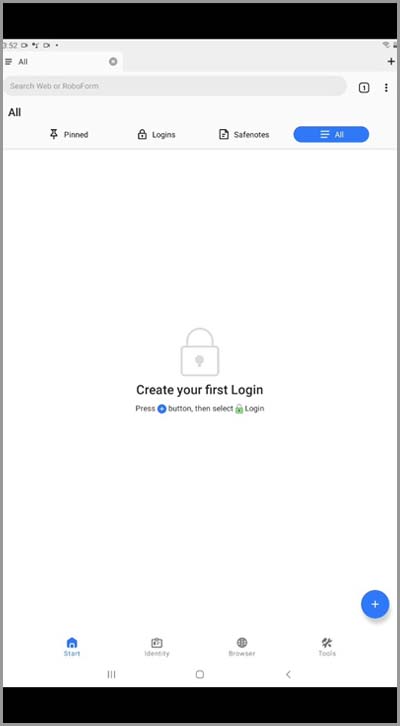The image is a screenshot taken from a mobile phone, depicting what appears to be an app interface.

At the very top of the image, there is a solid black banner. Directly below this, blurry and small, is the time displayed as 3:52. Adjacent to the time, various icons are visible: on the right-hand side, there’s what seems to be a WiFi icon followed by a partially filled battery icon. To the left, there's an icon with three lines next to the word "ALL," and to the right of that is a circle with an "X" inside it.

Beneath the top bar, the screen shows a search bar labeled "Search Web" within a long, rectangular, oval-shaped area. Below this, on the left side, the word "ALL" is displayed, then there is a pin icon labeled "PIN." To the right, a lock icon with the text "Logins" is visible, followed by a paper icon labeled "Safe Notes." The highlighted blue button to the right says "ALL."

In the center section of the screen, there is a lock icon next to the bolded text "Create Your First Login." Following this instruction, the text "Press" is present beside a blue circle button labeled "Button," and it continues with "then select" accompanied by another lock icon.

The area below features four icons, one of which appears to be a house, while the other three are less distinguishable. There's also a blue circle with a plus sign in it.

At the bottom of the screen, there are three icons: three horizontal lines, a square in the middle, and an arrow pointing to the left.